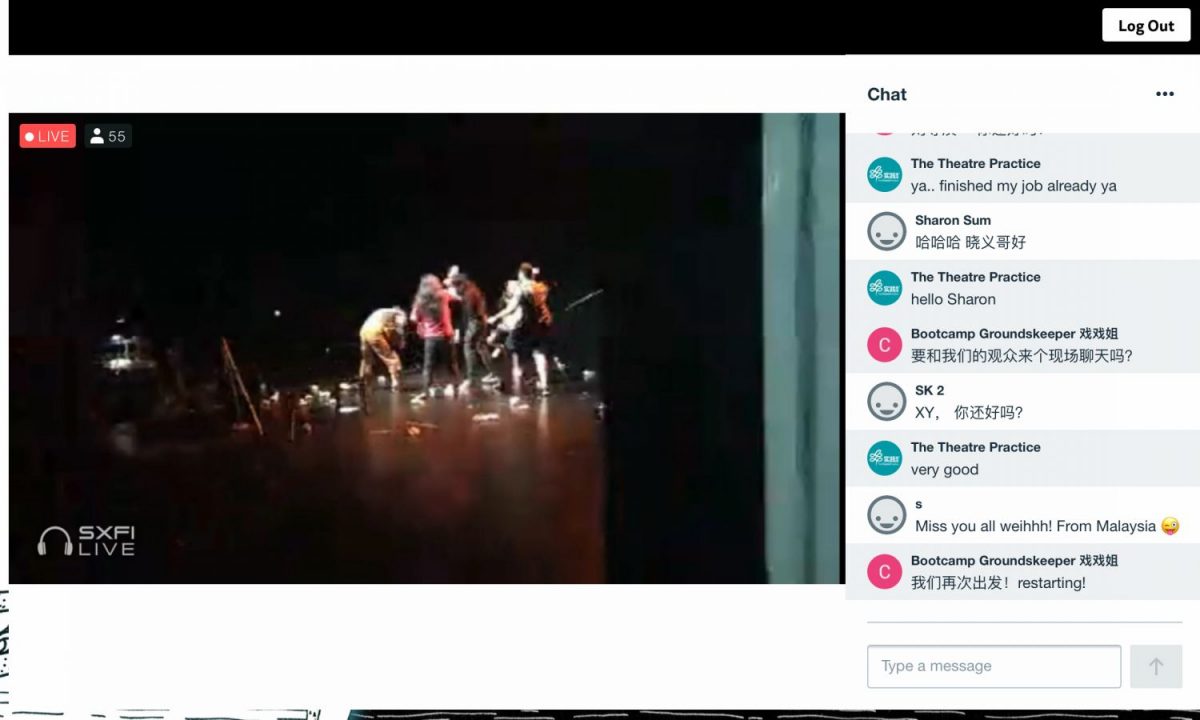A screenshot from a webpage capturing a live-streamed performance. 

Dominating the top section is a long, black, rectangular bar, with a white "Log Out" button positioned at the upper right corner. Below this bar, centered on the left, is a live-stream window showcasing an ongoing performance. The performance window is flanked by green curtains visible on the right side. A red button with a white dot and the word "LIVE" indicates the streaming status, with a white silhouette and the number "55" signifying the current viewer count.

At the bottom of the performance window, an icon of headphones accompanies the text "SXFI Live." The stage, primarily dimly lit in black, reveals five performers in action. On the right side of the image, a live chat interface is visible, providing a place for viewer interaction.